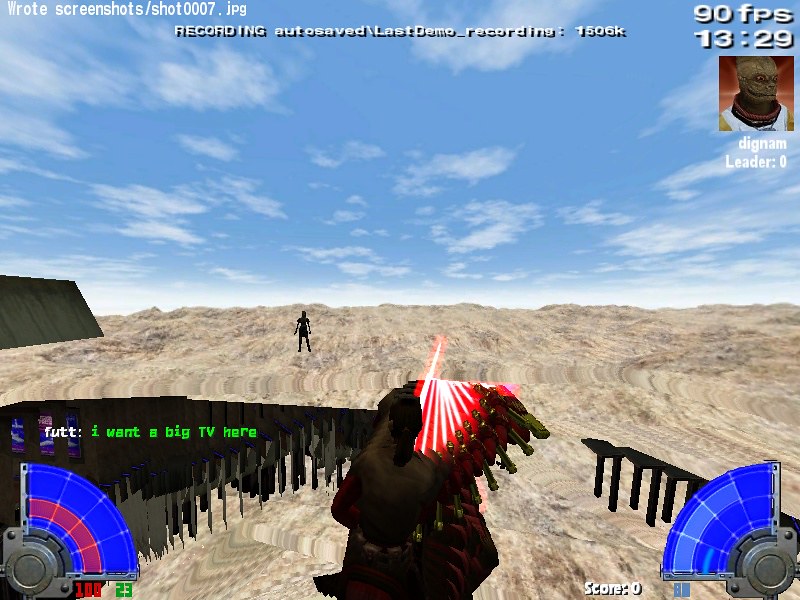In this detailed screenshot of a video game, various in-game and overlay elements are clearly visible, offering insight into both the game environment and some system metrics. The screenshot features a minimalistic first-person shooter (FPS) interface that appears quite rudimentary and basic in design. This stripped-down aesthetic emphasizes functionality over elaborate graphics.

At the top left corner of the screenshot, there is a visible watermark text, “wrote screenshot/shot0007.jpg,” indicating the file name or the saving process of the screenshot. Directly below this watermark, another string of text reads, “last recording auto saved last game recording = 1606K,” which likely refers to the size of the most recent automatically saved game recording, quantified as 1606 kilobytes. 

On the top right, performance metrics are displayed, including “90 FPS,” denoting the game's frame rate of 90 frames per second, ensuring smooth gameplay. Next to this, the number “1329” is displayed, which is presumably the current in-game time.

At the center of the interface, a name “Dingham” appears, which is probably the player's username. Indicated next to this name is “the leader: 0,” suggesting that Dingham is currently in the lead with no points or significant interaction yet, emphasizing the early and bare-bones state of the gameplay.

The visuals confirm the bare-bones nature of this game. The interface and environmental textures are basic, focusing mostly on essential elements without extensive graphical detail. This likely offers a straightforward and unembellished gaming experience, characteristic of early FPS games or newly developed indie projects.